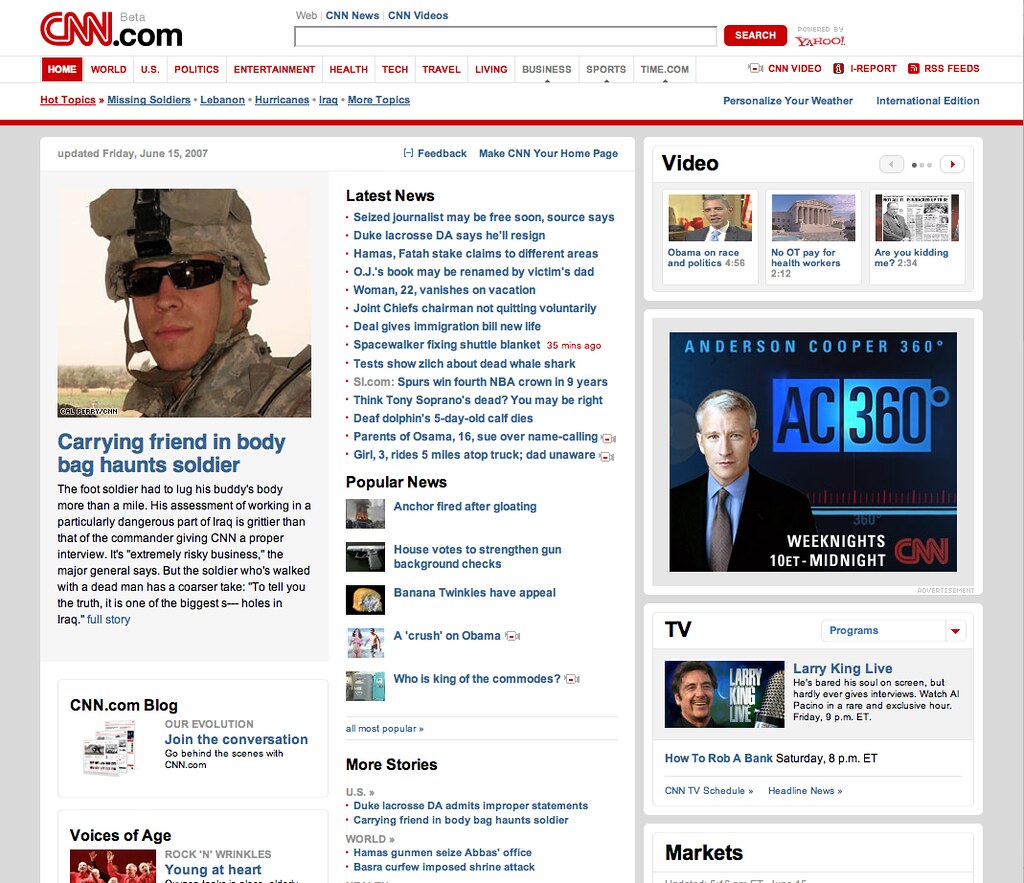**Caption:**

Website: CNN.com (Beta)

The webpage prominently displays "CNN" in bold red letters and ".com" in black. Above the logo, the word "Beta" is featured, indicating it's a test version. A search bar is located at the top, enclosed within a red box with the word "Search" in white letters, and it is noted to be "Powered by Yahoo." 

Navigation tabs are listed horizontally beneath the search bar, with "Home" highlighted in red with white text, followed by sections in red letters: "World," "US," "Politics," "Entertainment," "Health," "Tech," "Travel," and "Living." "Business" and "Sports" are displayed in black letters, with "Time.com" adjacent. 

A button labeled "CNN Video" precedes a menu for "Hot Topics," which lists currently relevant issues such as "Missing Soldiers," "Lebanon," "Hurricanes," "Iraq," among others.

A central image features a soldier wearing sunglasses and a helmet, with a caption stating: "Carrying friend in body bag haunts soldier," leading into an article on the topic. 

A sidebar titled "Latest News" includes headlines such as "Seized journals may be free soon," "Duke Lacrosse D.A. says he will resign," "Hamas- FATA state claims in different areas," and "OJ's book may be renamed by victim's dad."